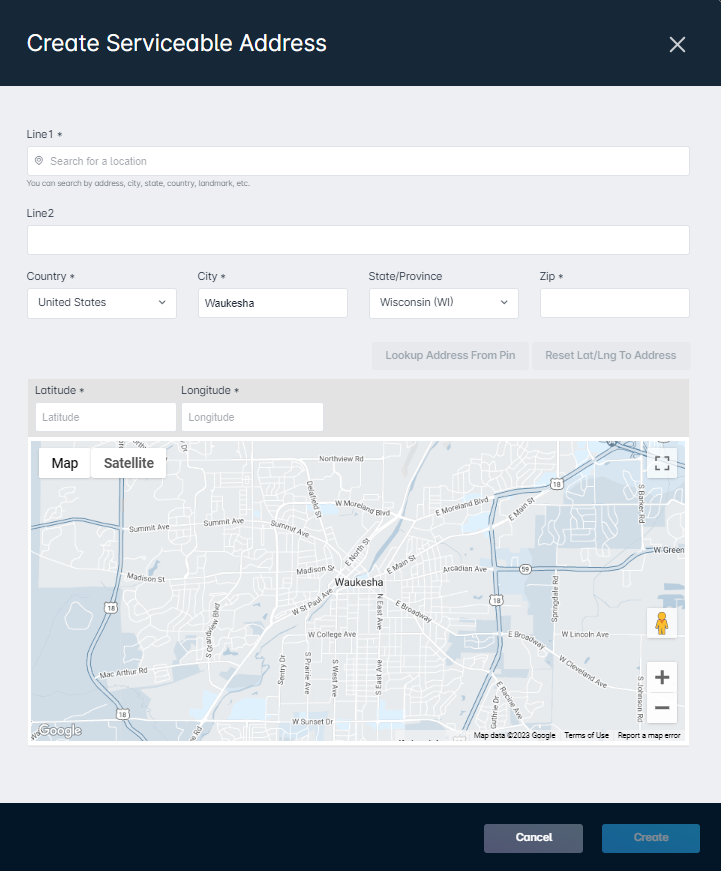**Detailed Caption:**

A website interface titled "Create Serviceable Address" displays several interactive fields for user input. At the top left, the title is presented in white text. To the right of this title is an 'X' symbol, allowing users to exit this section. 

Below the title, there is a search bar labeled "Search for a location," where users can input details such as address, city, state, country, or landmark. This search functionality is followed by a blank field on the second line, which currently holds no information.

Further down, there is a section divided into four parts for entering detailed address information: a drop-down menu for selecting the country (defaulting to the United States), a text box for the city (presently filled in with "Waukesha, Wisconsin"), and a field for selecting the state or province. The zip code field, marked with an asterisk to indicate it is mandatory, is currently empty. 

Additional options are provided beneath this: a button labeled "Lookup address from PIN" under the state/province field, and another labeled "Reset lat and longitude to address" under the zip code field. 

Below these functions, there are side-by-side text boxes for entering latitude and longitude coordinates. 

A map of Waukesha, Wisconsin, occupies the main section of the interface. At the top left of the map, users can switch between 'Map' and 'Satellite' views. On the top right, there are controls for zooming in and out, including a yellow stick figure icon for enabling street view. 

At the bottom of the page, a 'Cancel' button is highlighted in white, while the 'Create' button is dimmed, indicating it is not currently clickable.